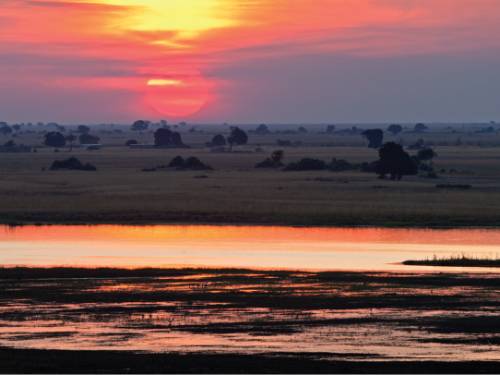This photograph captures a breathtaking sunset over the African safari landscape. The enormous, brilliant red Sun dominates the horizon, partially shrouded by clouds that create dramatic hues of purple and blue. The expansive sky transitions from a golden yellow at the top through vibrant oranges and reddish-pinks, culminating in a mesmerizing display of color. Below this vivid sky lies a vast flatland, characteristic of African grasslands, interspersed with sparse, dark silhouettes of trees. In the mid-ground, a green field dotted with shrubs and additional trees stretches out, giving way to a low-lying marshy area with some scattered weeds. This wet, marsh-like section appears to reflect the striking colors of the sky above, enhancing the scene with a mirrored orange glow. The overall composition presents a serene yet dynamic environment, capturing both the tranquility and raw beauty of the safari at sunset.